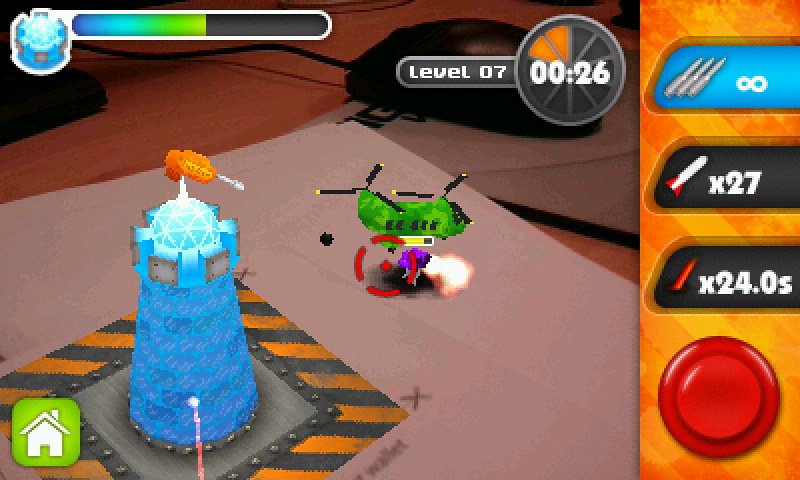This screen capture from a video game portrays an intense moment of action. A blue tower mounted on a small platform, equipped with an orange gun, takes aim at a formidable green helicopter with dual propellers. Below the helicopter, a nearly full yellow energy bar—indicating about 80% capacity—and a small red target marker emphasize the ongoing battle. The ground surface resembles a piece of paper, over which an explosion manifests as a swirl of purple smoke, enveloping the scene in chaos.

The blue tower sits within a caution-marked perimeter, distinguished by thick black and yellow striped borders. A red laser beam emanates from this tower, extending to the bottom of the screen. On the lower left, a green button featuring a house icon designates the home menu. At the top of the screen, an energy bar for the tower, currently around 55% full, is displayed beside a tower icon. Beyond this paper-like battleground, in-game elements include a mouse pad and a mouse, adding a layer of meta-reality to this vivid scenario.